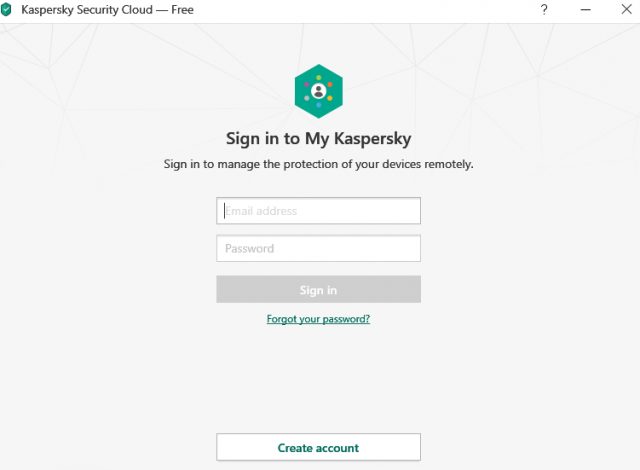Kaspersky Security Cloud: My Kaspersky Sign-In Page

The image depicts a minimalist sign-in page for Kaspersky Security Cloud’s “My Kaspersky” portal. The interface is clean, with a light gray background accented by a few green elements. The Kaspersky logo is simple, resembling a head and upper torso within a green hexagon, akin to a default user icon.

In the center of the page, users are prompted to sign in by entering their email address and password. Below the input fields is a prominent Sign-In button. Additional options include a “Forgot Your Password?” link and a “Create Account” button, both located at the bottom of the page.

The windowed design allows users to minimize or exit the page, and a question mark button is available for assistance. This interface enables users to manage the protection of their devices remotely.

Note: Due to allegations of Kaspersky’s close ties with the Russian government, users might want to exercise caution when considering the use of this service.